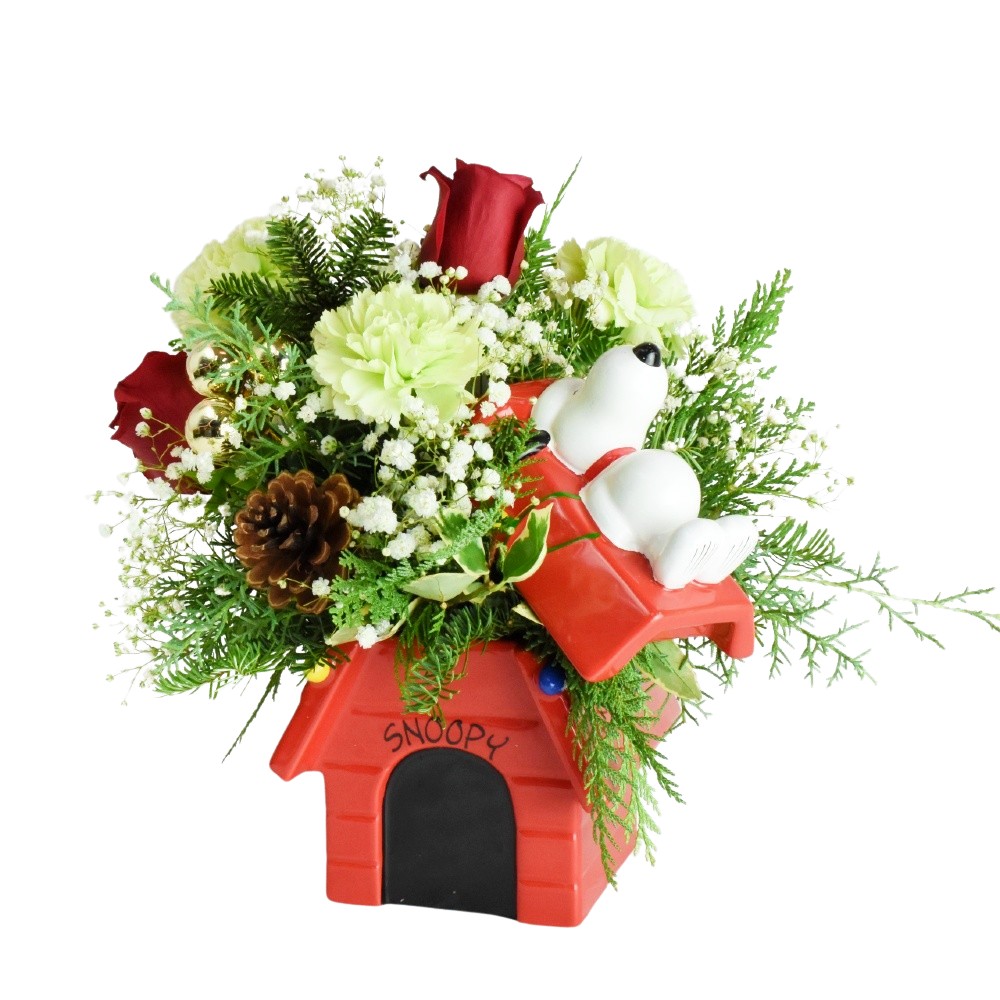The image showcases a charming, festive arrangement featuring Snoopy's iconic red doghouse, adorned with the name "Snoopy" in black text on the front. On top of the doghouse, Snoopy, the beloved character from Charlie Brown, is seen resting in a small bed-like space as part of the composition. This delightful setup is integrated into a winter-themed flower bouquet that includes vibrant red roses, delicate white carnations, petite white baby's breath, and lush greenery, accented with a rustic pine cone. The ornament exudes a glossy, smooth finish, suggesting materials like glass or plastic, enhancing its festive appeal. This piece would make a lovely holiday gift or a charming addition to a hallway table, embodying the spirit of Christmas with its cheerful design and seasonal flowers.